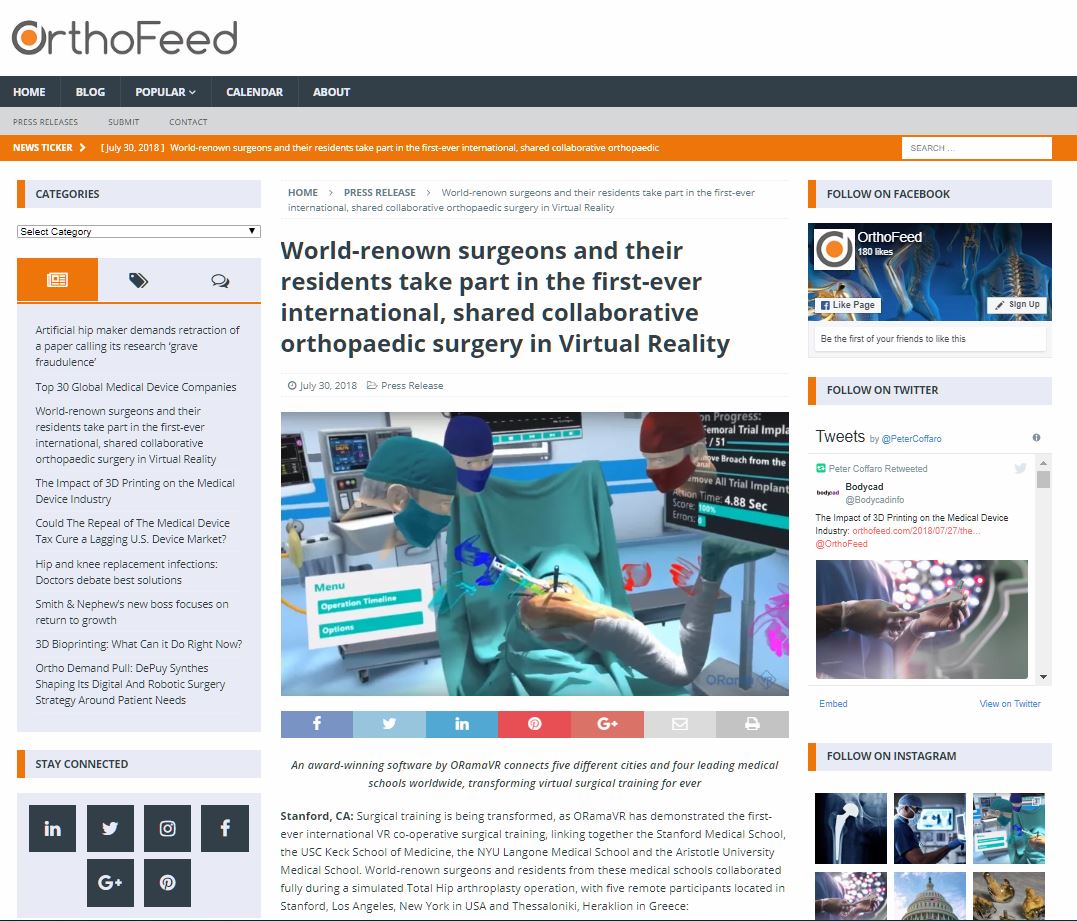The image showcases the OrthoFeed website, prominently displaying its logo on the upper left-hand side above a dark green-gray horizontal navigation bar. This bar features left-justified menu options including Home, Blog, Popular, Calendar, and About. Just below this, a secondary light gray menu offers options for Press Release, Submit, and Contact.

At the center of the webpage is an article titled, "A World of Renowned Surgeons and Their Residents Take Part in the First-Ever International Shared Collaborative Orthopedic Surgery in Virtual Reality." Directly below the article title is an accompanying image that features three virtual doctors engaged in a surgical procedure. The doctors are wearing masks and TED hair protectors, fully immersed in a virtual reality environment for the groundbreaking collaborative surgery.